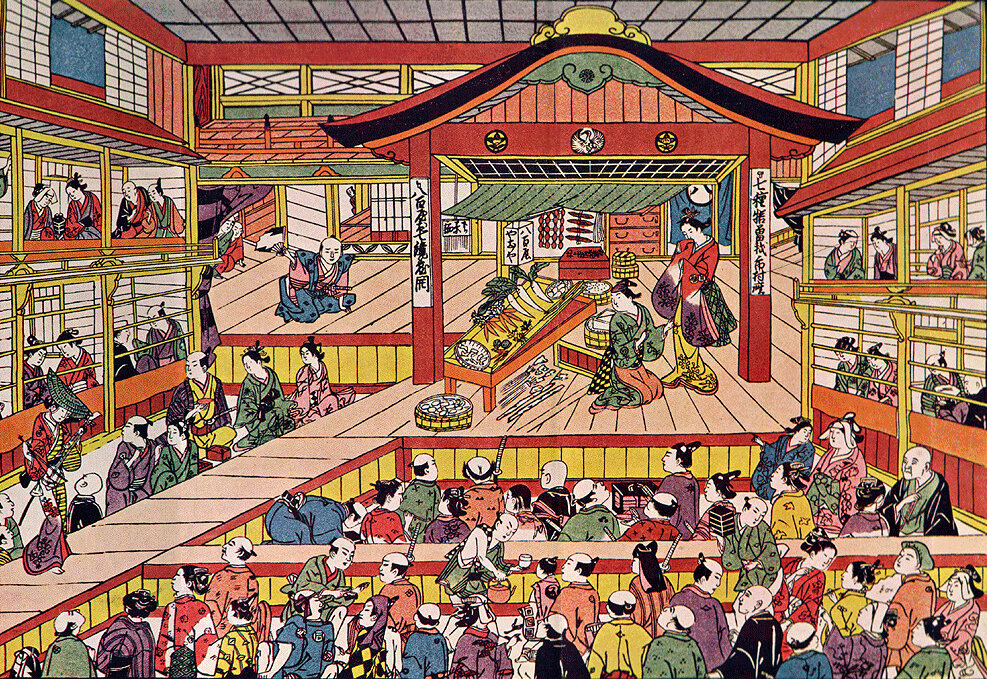The image in front of me is a richly detailed, multicolored historical drawing, possibly from a Japanese or Asian dynasty, depicting a bustling market scene or perhaps a celebration. The predominant colors in this intricate artwork are vivid shades of red, light pink, yellow, green, and orange. 

In the center of this crowded composition, there is a stage where several geisha women are prominently featured. On this stage, three women are organized around a table adorned with various fruits and vegetables. One woman is tending to the table, while another holds a sack, and a third woman kneels down. The floor of the stage has a peach hue, and the scene appears to thrive with cultural significance and traditional attire.

Surrounding the stage, numerous figures walk along a large floor space, engaging in conversations and moving about with a sense of activity and liveliness. They all seem to be participating in what looks like a vibrant market atmosphere, enriched by platforms on either side of the central stage. These platforms, resembling multistoried structures with bar-like railings, also host a multitude of people, enhancing the crowded, dynamic nature of the scene.

The image is meticulously drawn with a celebratory feel, capturing the essence of an old-fashioned public space suffused with historic and cultural elements. Small details like side rooms above the stage, where more individuals are positioned, add to the complexity, making this a vivid depiction brimming with narrative and color.